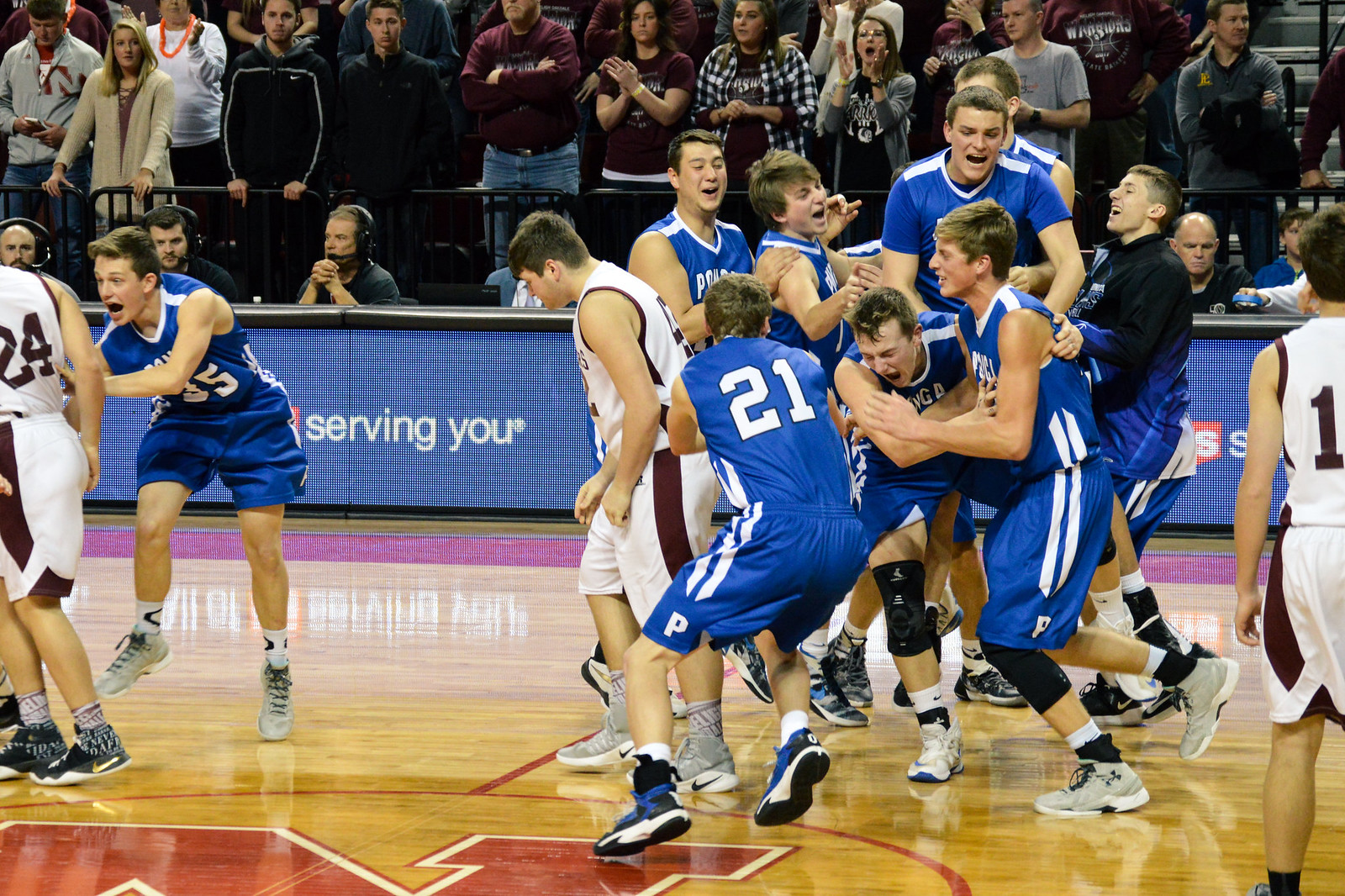This detailed sports photograph captures the climactic moment of a high school basketball game, likely held during the Nebraska State championships or playoffs, given the prominent red letter "N" visible on the court floor, potentially representing the University of Nebraska. The image shows a jubilant team in royal blue jerseys with white numbers and stripes, some featuring a "P" on their shorts, celebrating their victory. Many of the blue team players are clustered together in a joyful embrace, with others running towards them, all wearing low socks and a couple sporting knee protectors. In stark contrast, the opposing team in white jerseys with black or maroon stripes and numbers, including a visible number 24, stands dejected on the court. In the background, the crowd's reaction mirrors the teams' emotions. While only a few fans appear to be clapping supportively, the majority, likely rooting for the white-jersey team, look disappointed. The court itself has a distinctive brown tile appearance, and along the sidelines, there's a waist-high wall with blue siding and a black top, bearing part of the text "serving you." This horizontally aligned image vividly captures the contrasting emotions of triumph and defeat in high school sports.